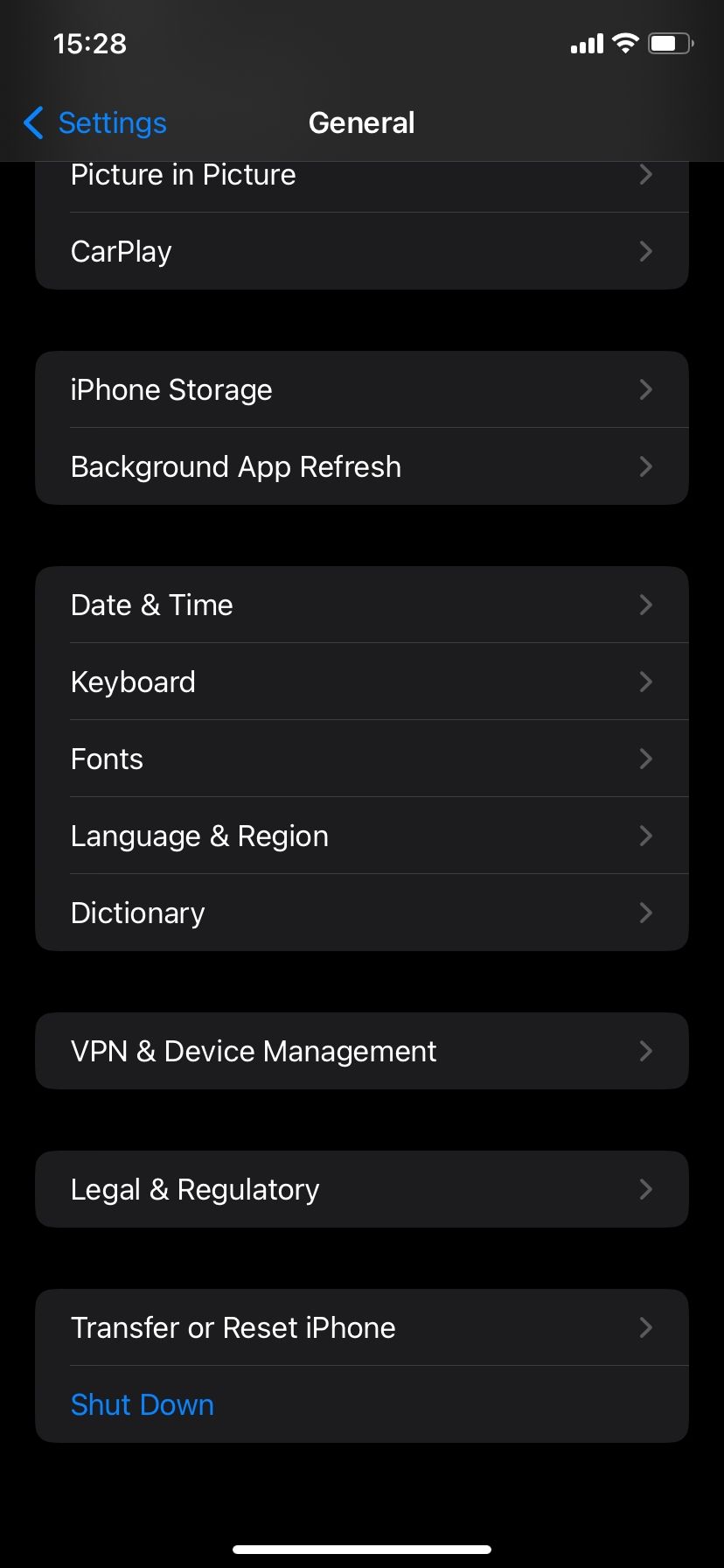The image is a screenshot taken from a cell phone with a black background. At the top, the time "15:28" is displayed in white font, alongside a battery bar, a network logo, and a Wi-Fi icon, all in white. The screenshot showcases the settings menu, identifiable by a blue back arrow and the word "Settings" also in blue. Centrally positioned at the top is the section title "General" in white text. Below this title, a list of options are present, each accompanied by a right-pointing arrow, all in white text. The options include "Picture in Picture," "CarPlay," "iPhone Storage," "Background App Refresh," "Date & Time," "Keyboard," "Fonts," "Language & Region," "Dictionary," "VPN & Device Management," "Legal & Regulatory," "Transfer or Reset iPhone," and finally, "Shutdown" in blue text.